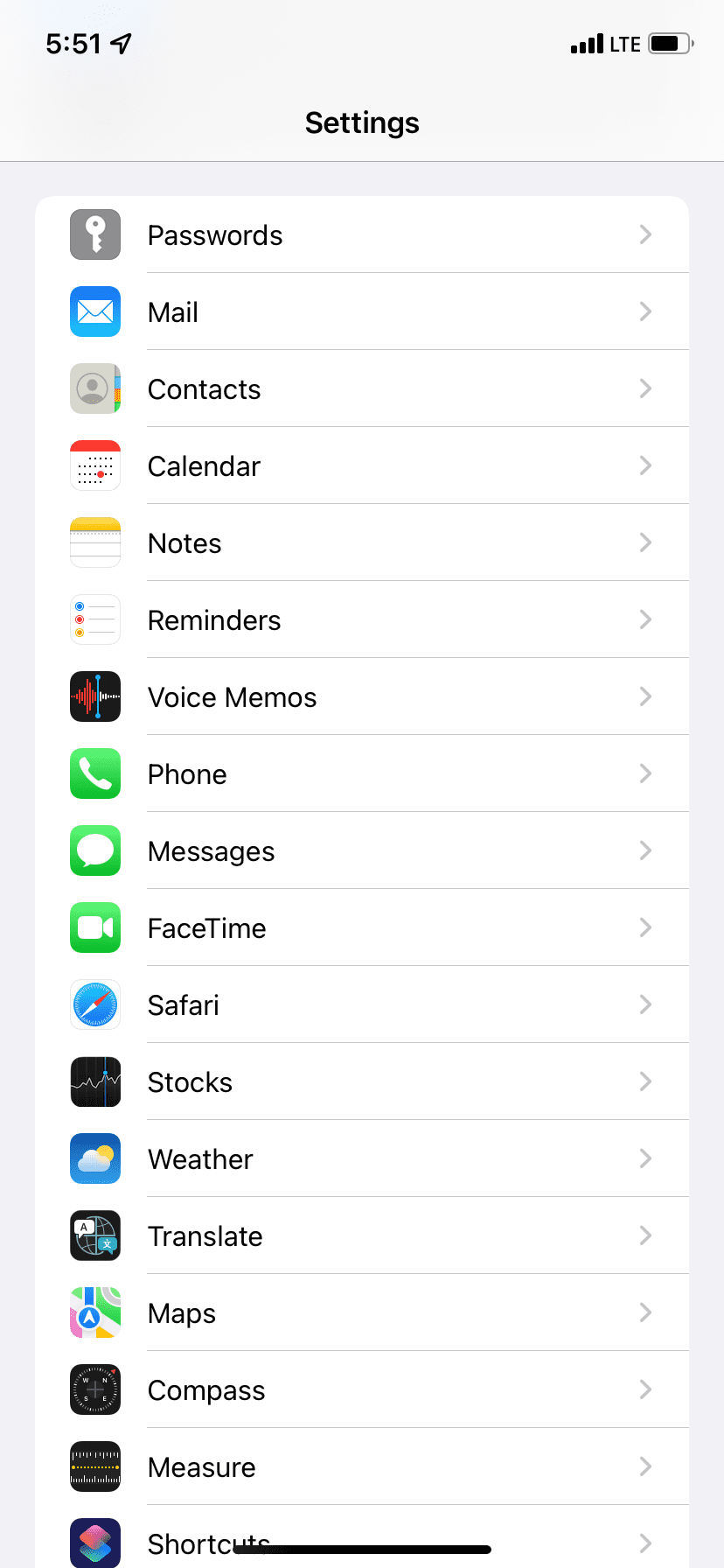The image appears to be a screenshot from a mobile phone displaying a settings menu. The background is predominantly white with a grey band framing the top and sides of the screen. A thin horizontal line extends a third of the way across the bottom of the display, intruding slightly into the text.

At the very top left corner, the time is shown as 5:51 alongside a small arrow icon. The top right corner displays standard mobile status icons, including LTE signal strength, and a battery icon. Centrally located at the top is the word "Settings."

The list below details various settings categories, each accompanied by an icon and a right-facing arrow:

1. **Passwords**: Represented by a grey box containing a white key icon.
2. **Mail**: Displayed with a blue box featuring a white envelope icon.
3. **Contacts**: Indicated by a grey icon.
4. **Calendar**: Shown with an icon resembling a calendar, highlighted with a red top.
5. **Notes**: Depicted as a notepad with a yellow top.
6. **Reminders**: Marked by three colorful bullet points.
7. **Voice Memos**: Illustrated with a sound file image in black.
8. **Phone**: Represented by a white phone icon on a green background.
9. **Messages**: Shown as a green message bubble icon.
10. **FaceTime**: Depicted as a white video recording camera on a green background.
11. **Safari**: Identified by a blue circle icon.
12. **Stocks**: Displayed with a small graph on a black background.
13. **Weather**: Represented by a cloud and sun icon on a blue background.
14. **Translate**: Shown as a white and blue rectangle on a black background.
15. **Maps**: Exhibited as a multicolored map icon.
16. **Compass**: Shown as a tiny icon on a black background.
17. **Measure**: Also depicted with a tiny icon on a black background.
18. **Shortcuts**: This icon, partially obscured by the bottom line, is a rounded blue and pink icon on a black background.

The detailed and precise icons and labels provide clear indications of the various functional settings available on this mobile device.